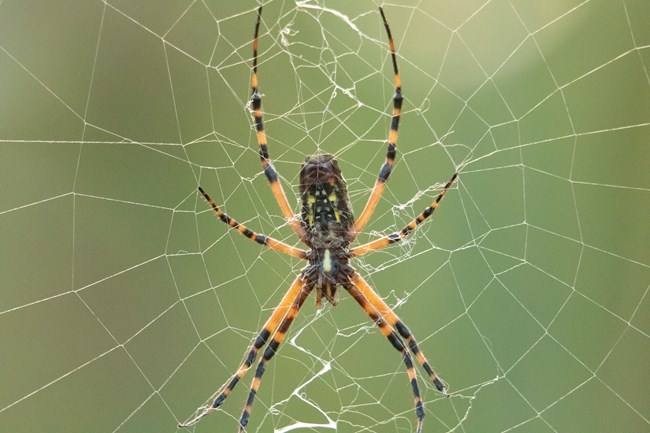In this detailed rectangle-shaped photograph, a large spider takes center stage, meticulously crafting its web against a blurred background of muted pea green that gradually lightens to a yellowish-white on the top right. The spider, the main focus of the image, is suspended in the middle of an intricate web, which starts with a circular formation of white silk strands radiating outward. As you move closer to the spider, the web transitions into a chaotic zigzag pattern, seemingly emanating from the spider itself, hinting at the ongoing web-building process. The spider boasts a brownish-black body with alternating orange and black striped legs, where the black spots are more pronounced towards the tips. Its vibrant coloration and detailed webbing create a striking contrast against the soft, green backdrop, emphasizing both its delicate beauty and the intricacy of its natural craftsmanship.